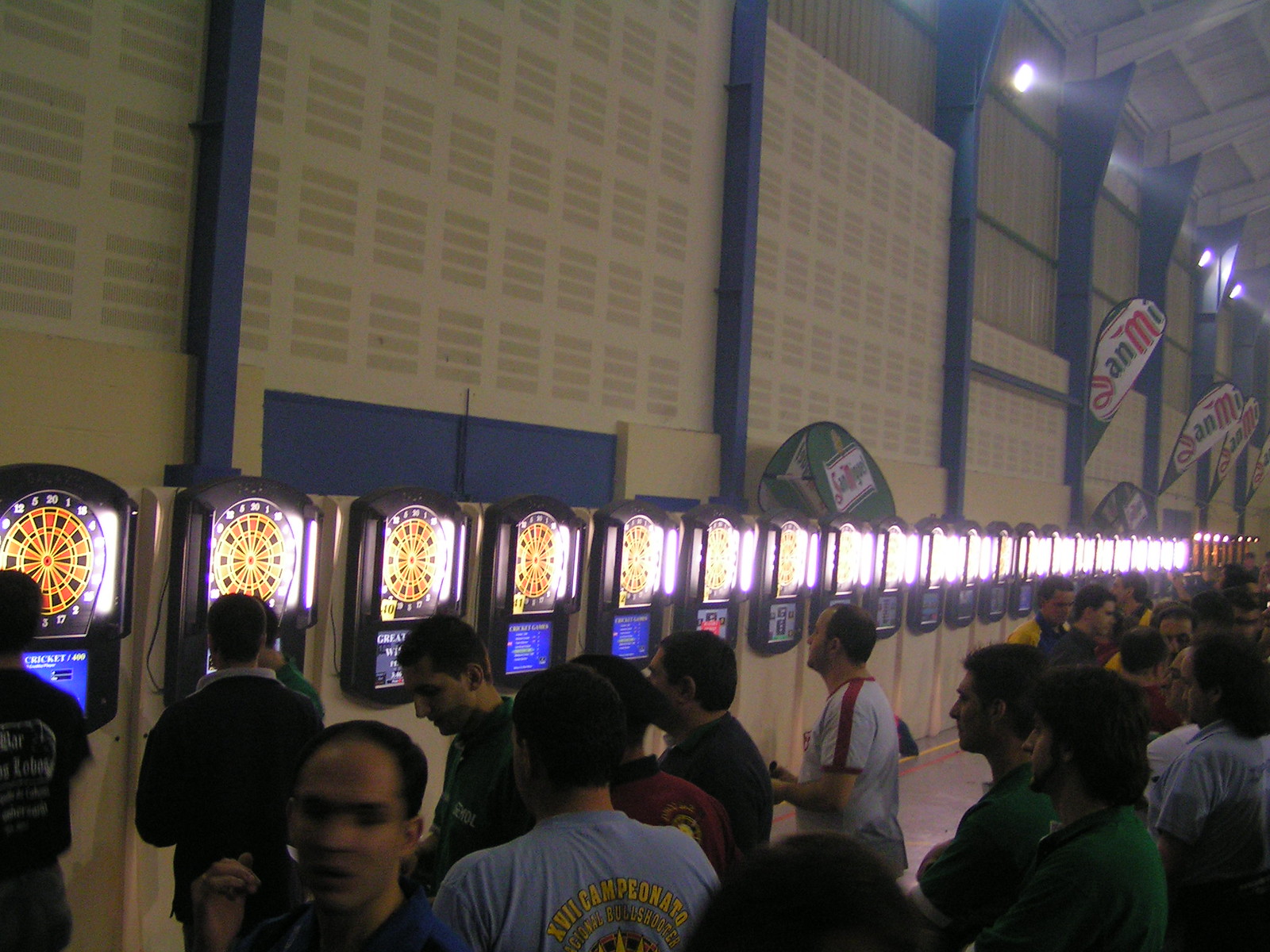The photograph depicts a bustling, possibly Asian-majority crowd inside a large, warehouse-like structure. The space, which could be a sports complex or a casino, features a long row of digital dartboards lining a beige wall with black vertical posts. Each dartboard is backlit and topped with monitors that display blue screens, some of which are illuminated. The high ceiling is supported by beige rafters, and overhead lighting is present.

In the foreground, many people are interacting with the dartboards, holding various items such as phones or betting slips, and appearing to be engrossed in the activity on the screens. The room's expansive, two-story tall layout is reminiscent of a gymnasium or expansive casino hall, with its dim lighting punctuated by the glow of the dartboards. The detailed setup and lively crowd suggest that this is a popular, possibly competitive venue.